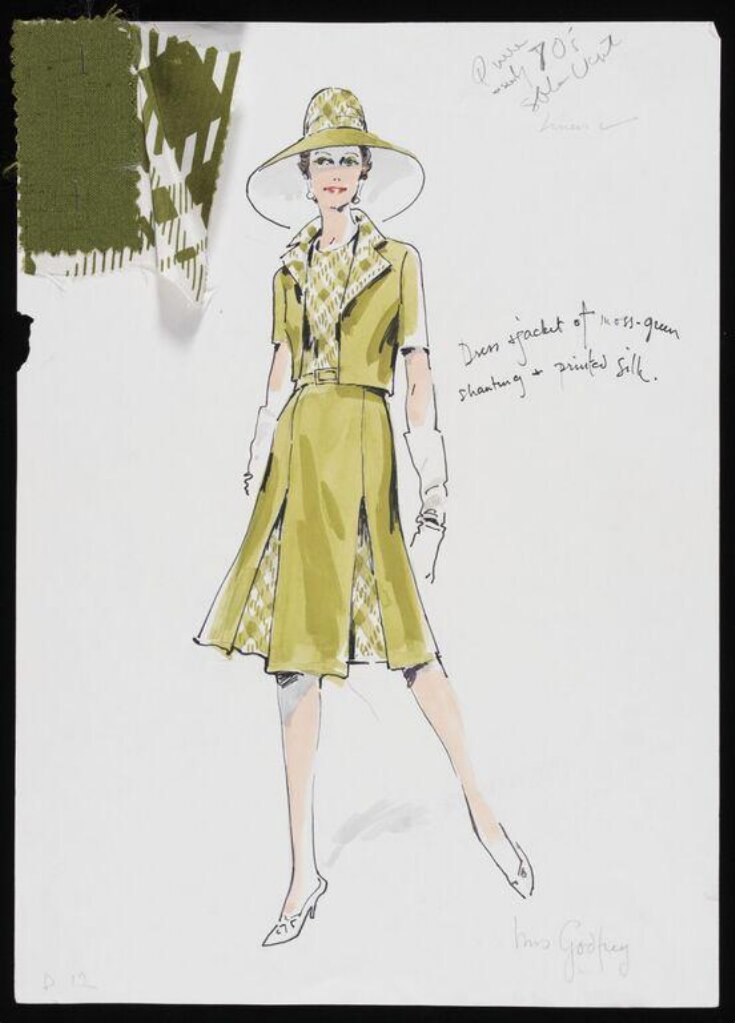This color illustration, resembling a fashion designer's quick pen and ink sketch, showcases an elegant women's outfit prominently in a vertical, portrait-oriented frame with black edges. The model, gazing upwards, dons a wide-brimmed hat from the 1950s era, featuring a gold color with a gold plaid pattern on top and white underneath the visor. Her sophisticated attire includes a short-sleeved dress jacket in moss green, made of shantung and printed silk, with a turn-back collar accentuated by a matching gold plaid. Beneath the jacket, she wears a gold plaid shell top, and her knee-length pleated skirt displays the gold plaid inside the pleats, matching the jacket and hat. Complementing the ensemble, she's adorned in white evening gloves, low-heeled white shoes, and holds a small bag. Detailed handwritten notations and a faint designer's autograph, likely "Godfrey," appear in the lower right corner. On the upper left, two fabric swatches – an olive green and a green and white plaid – are attached, providing a tactile sense of the materials used in this stylish creation, all set against a white, slightly torn background.